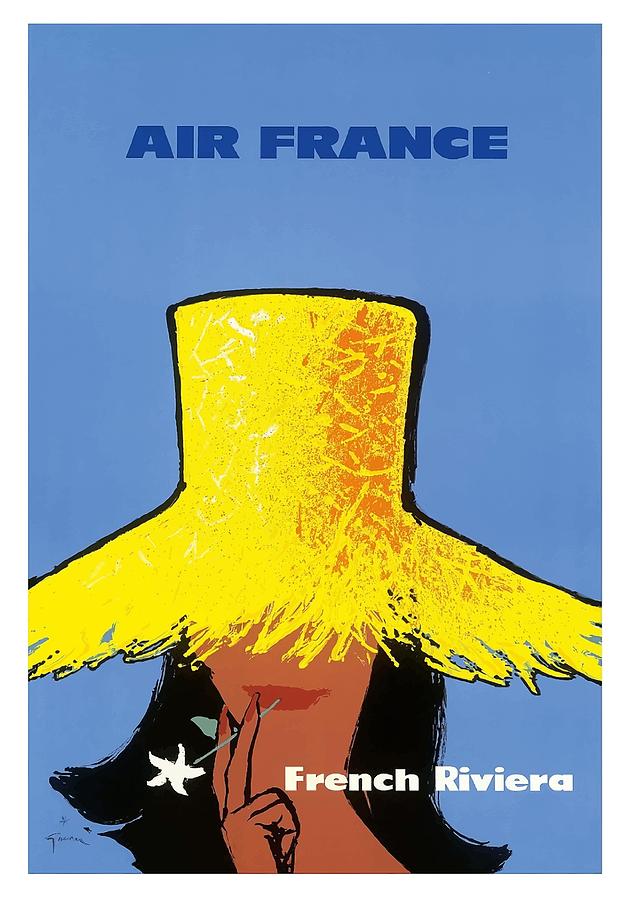This travel poster, predominantly rendered in light blue, prominently features the text "Air France" in dark blue at the top and "French Riviera" in white at the bottom right. Central to the illustration is a sophisticated woman with dark brown skin and shoulder-length, flipped-up black hair. She dons a striking, oversized straw hat, golden yellow in color, with a dramatically wide and low brim that largely conceals her eyes, allowing only her red lips to be visible. The hat's brim is irregular and shaggy, resembling torn straw. The woman's fingers are elegantly poised near her lips, holding a white flower with a light green stem, reminiscent of a cigarette. This composition creates an alluring and stylish impression, encapsulating the exotic charm of the French Riviera.